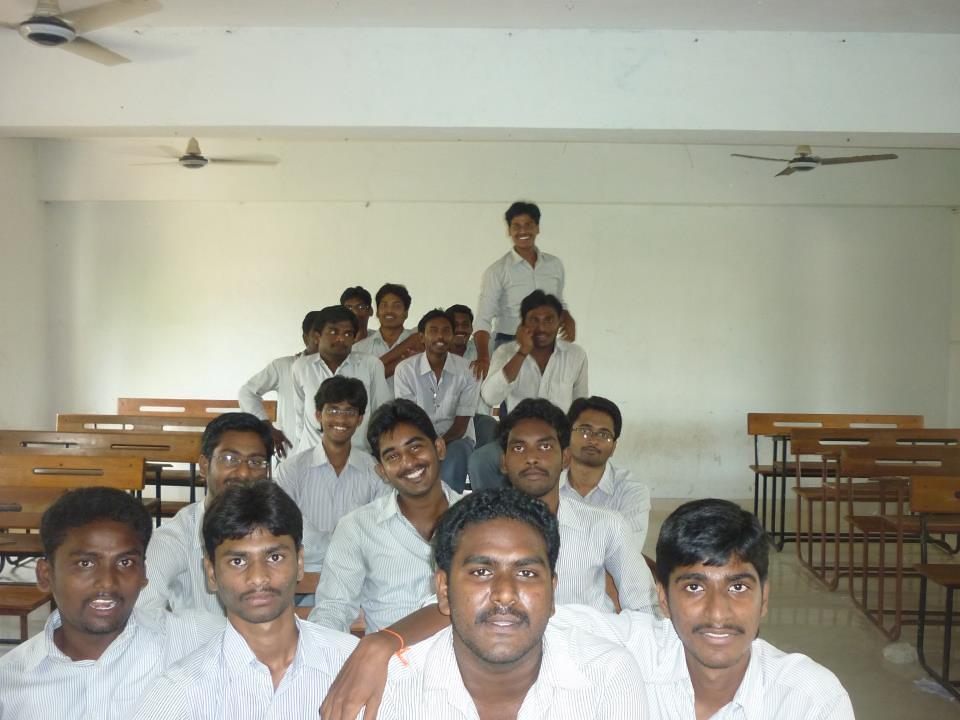This photograph captures approximately 15 men of Indian or possibly African descent, all with short black hair and dark skin, sitting or standing in what appears to be a white-walled classroom. Arranged in a triangular formation, the front rows are seated, the middle rows are perched on desktops, and one man stands on a desk at the back. They all don long-sleeved, white shirts with thin blue or gray stripes. Smiling and looking directly at the camera, they exude a sense of camaraderie and happiness. The room is lit by daylight streaming through the windows, while three brown ceiling fans overhead suggest a warm environment. Wooden desks flank the group, reinforcing the classroom setting.